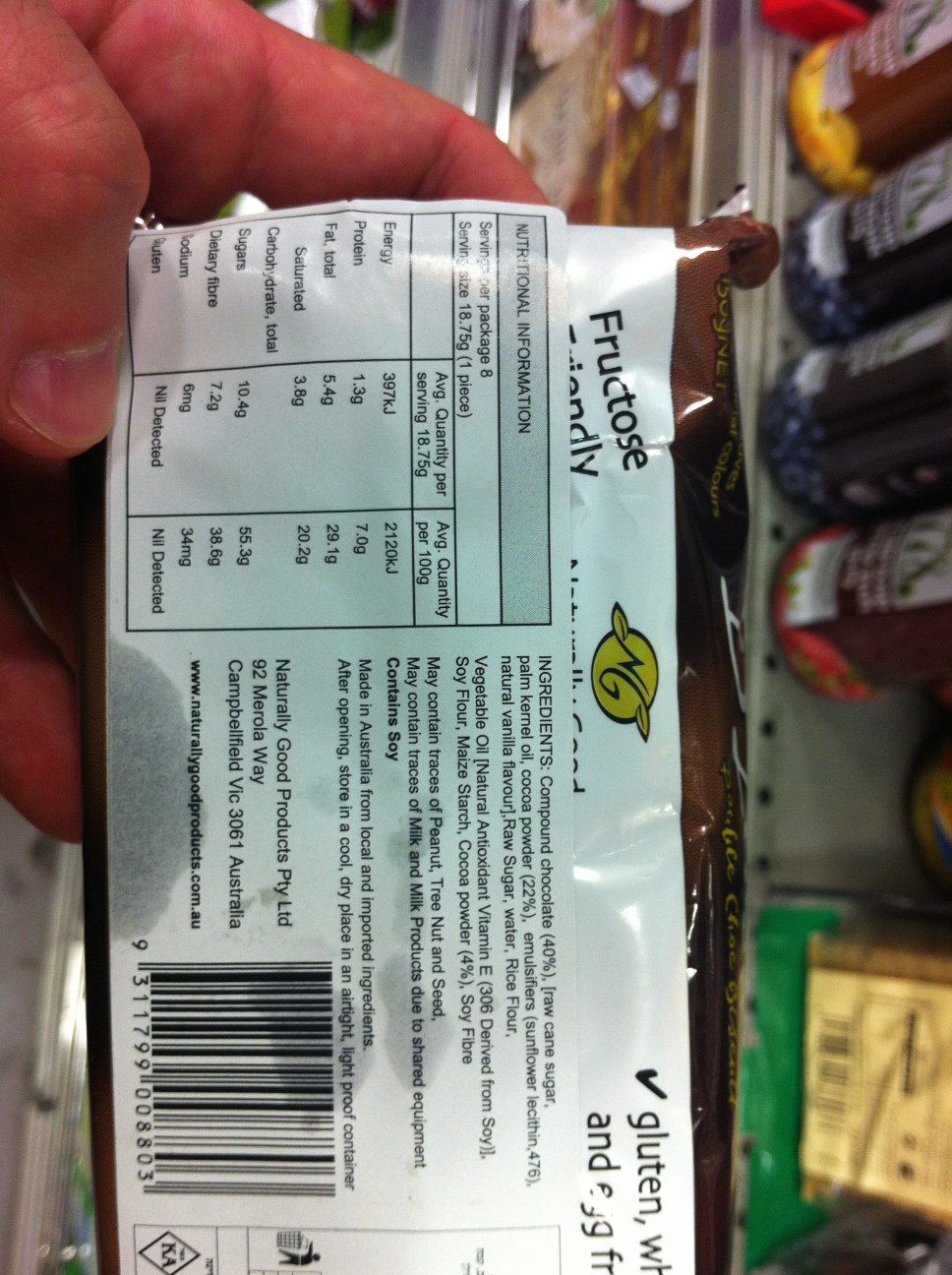In the image, a hand prominently holds a rectangular packaged food item, displaying the backside of its wrapper. This packaging is predominantly white and covered with black text, detailing nutritional information and a list of ingredients. A barcode is situated in the lower-left corner of the wrapper. In the blurred background, shelves stocked with various grocery items, which appear to include jars possibly containing jelly or jam, give context to the setting, suggesting the scene takes place in a store aisle. The composition focuses on the detailed text and minimalist design of the packaging, contrasting with the colorful and varied items behind.